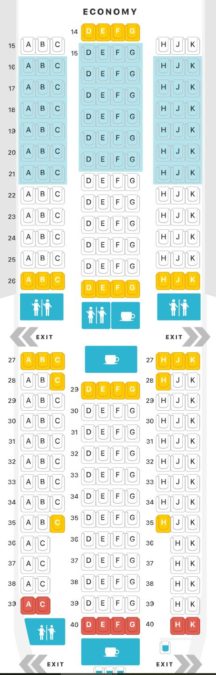This photograph depicts a Scantron sheet, commonly used for standardized tests. At the top, the word "Economy" is visible, which may indicate the brand or the subject matter of the test. The sheet starts at question 14, with possible answers labeled D, E, F, and G. 

The Scantron sheet is marked with various colors: questions 14–15 and 26 are highlighted in a yellow-orange color, while questions 16–21 are marked with a blue highlight. Question 39 has options A and C highlighted in red, and question 40 shows highlights from D to K, ostensibly indicating skipped answers or notes.

Additionally, blue icons featuring drawings of people appear at the bottom of the sheet. There are other sporadic highlights across the document, and an "EXIT" marking is also present. The highlights and markings seem to serve as a guide or indication for specific response actions.